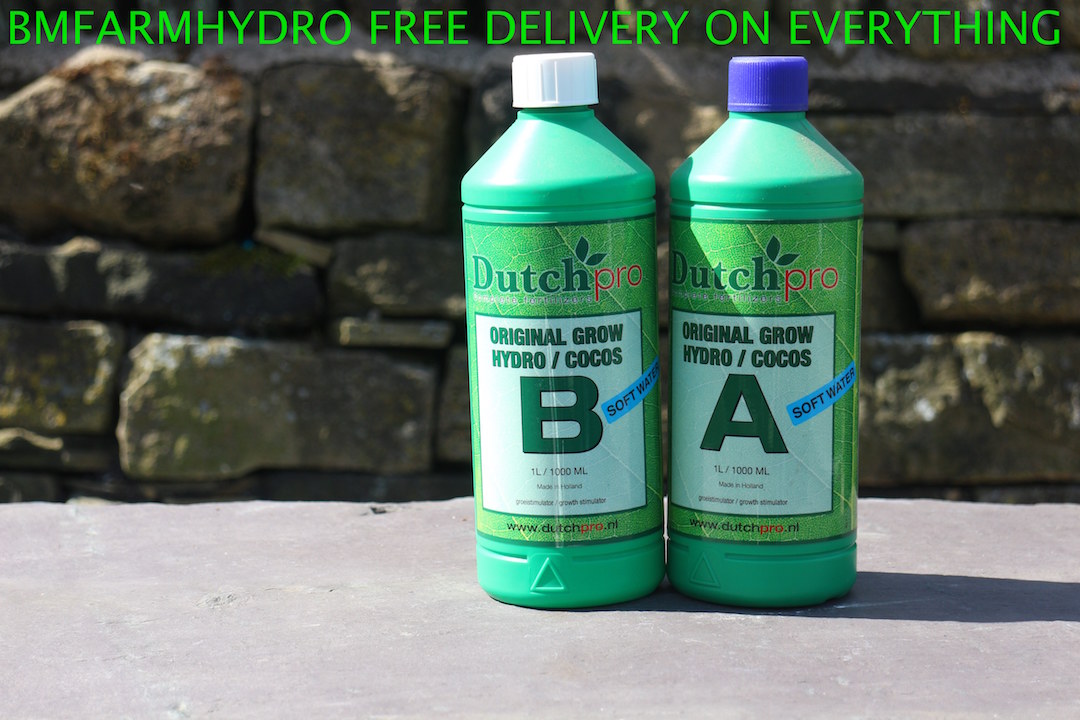This advertisement features a wide rectangular image showcasing two tall green bottles positioned slightly to the right of center on a gray cement horizontal surface. Set against a backdrop of large, unevenly sized gray bricks, the bottles prominently display bright green leaf stickers. At the top of these stickers, "Dutch Pro" is written, with "Dutch" in green and "Pro" in red. Both bottles feature a large white square; the one on the left reads "Original Grow Hydro / Cocos B" in bold green font, while the one on the right reads "Original Grow Hydro / Cocos A" in the same font. The "B" bottle is capped with white, and the "A" bottle with blue. Additionally, these products are marked with a diagonal blue sticker indicating "soft water" and are advertised as one liter bottles. Above the bottles, an all-caps green text highlights the brand "BM Farm Hydro" with a note of "free delivery on everything." This detailed composition effectively presents the advertised farm growing botanical products amidst a rustic, industrial setting.